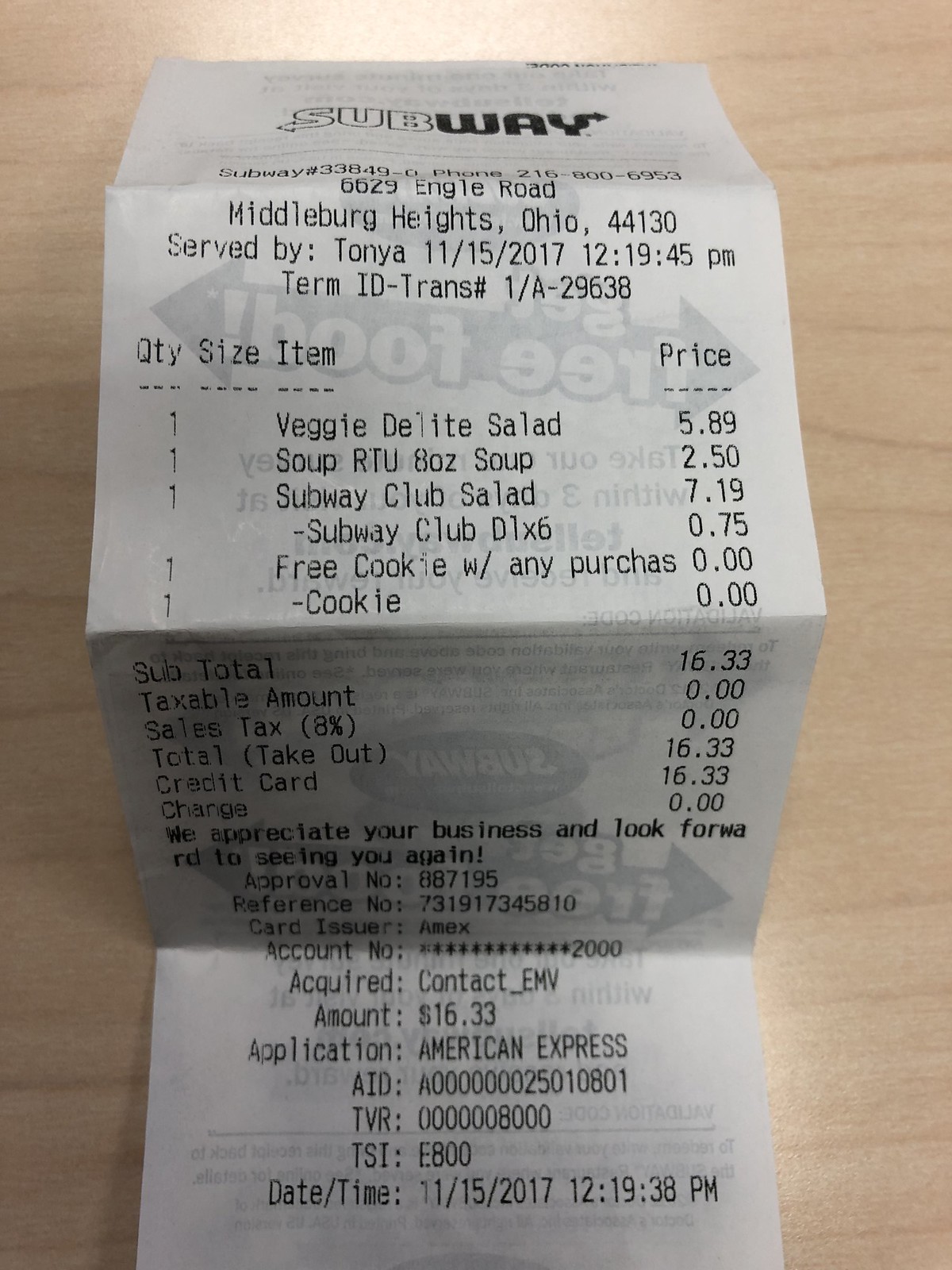This photograph captures a folded Subway receipt placed on a light wooden surface, possibly a desk or table. The receipt, predominantly in black and white, clearly displays the name "Subway" at the top. Below this, it provides specific location information: 6629 Engle Road, Middleburg Heights, Ohio, 44130. The receipt indicates that the server for this order was Tanya. The purchase took place on November 15, 2017, at precisely 12:19:45 PM.

A detailed list of ordered items follows: a Veggie Delight Salad, a soup, a Subway Club sandwich, and complimentary cookies with the purchase. The total amount for the transaction was $16.33, with no additional tax applied. At the bottom, the receipt notes that the payment was made using an American Express card. The receipt itself shows signs of having been folded multiple times, likely in quarters.